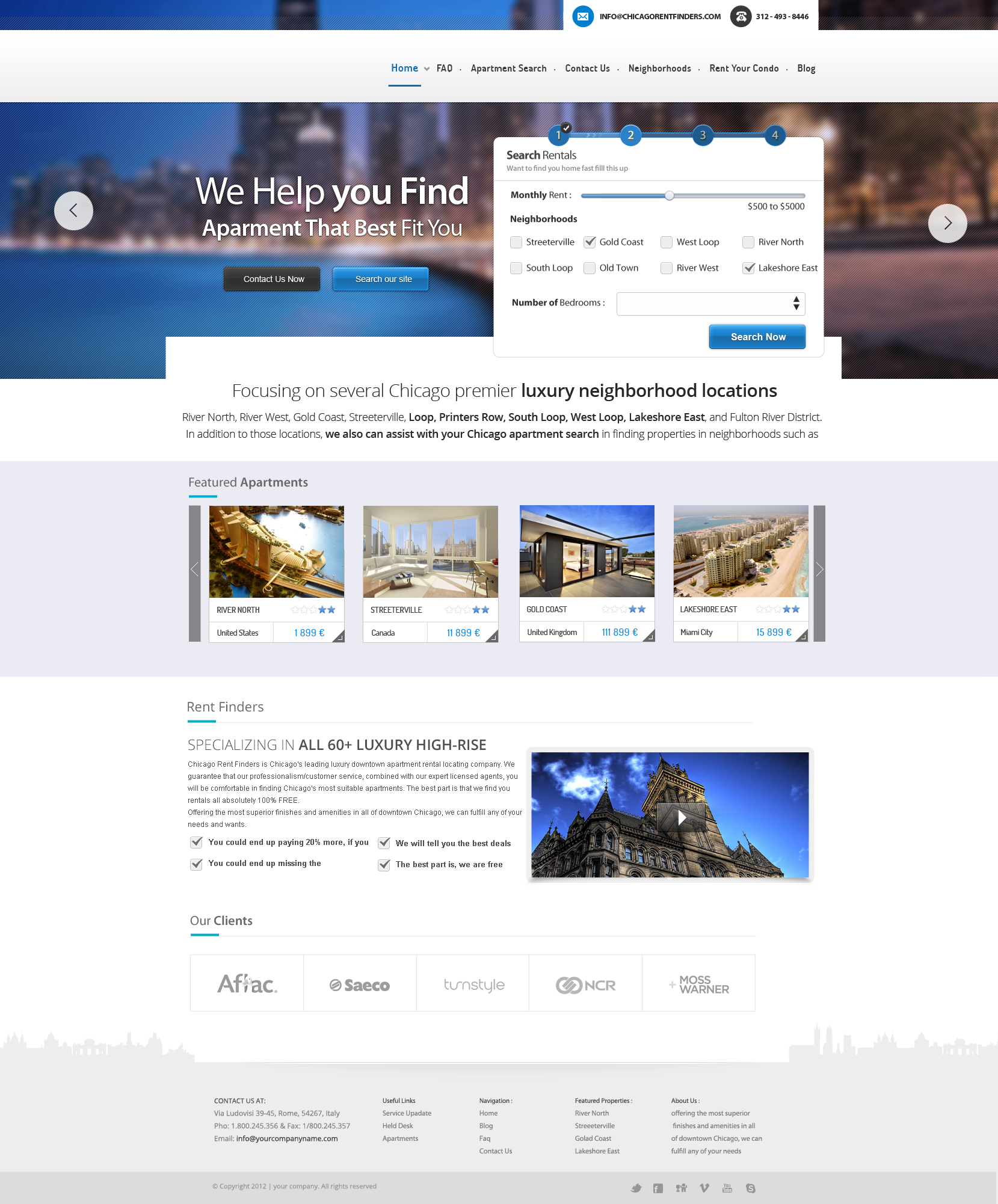The image depicts a webpage of an apartment search platform, "ChicagoRentSomething.com." The banner at the top prominently displays the tagline, "We help you find an apartment that best fits you." To the right of the banner, a user input section is visible where prospective tenants can fill in details such as monthly rent, type of neighborhood, and number of bedrooms. The background features a panoramic view of downtown Chicago, adding a distinctive urban feel to the site. Scrolling down, the page highlights featured apartments in several of Chicago’s premier luxury neighborhoods. This section lists various properties, though there seems to be a discrepancy with the pricing displayed in euros; one apartment is listed at 1,900 euros and another at 112,000 euros, likely indicating placeholder amounts. Further down, the site mentions "Rent Finders," which specializes in over 60 luxury high-rise apartment buildings.